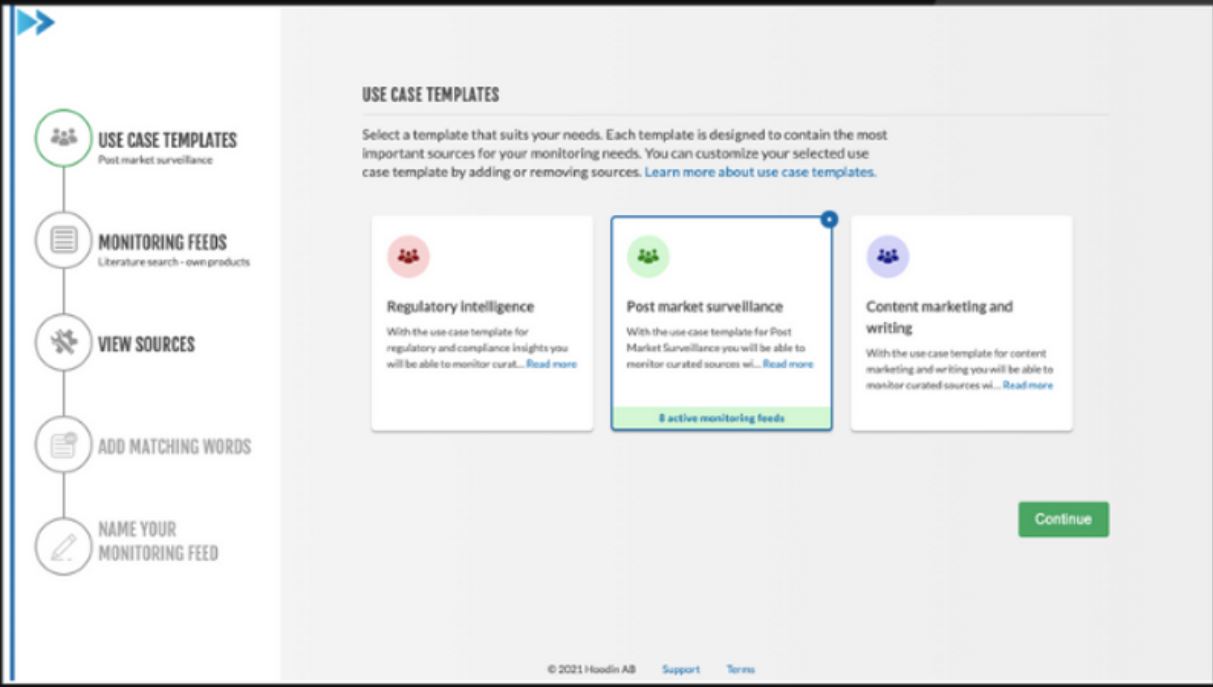This screenshot from a website features a complex user interface designed for use case templates. In the top left corner, two teal arrows point to the right, giving direction. Taking up the left-hand area is a white rectangular section filled with circles, each interconnected by gray lines, likely representing a workflow or process sequence. 

The uppermost circle in this white area is highlighted, indicating it has been clicked on. It depicts a group of three people and provides options titled: 'Use Case Templates,' 'Monitoring Feeds,' 'View Sources,' 'Add Matching Words,' and 'Name Your Monitoring Feed.'

To the right of this white section, a much larger, faint gray area dominates the screen. At its top, 'Use Case Templates' is prominently displayed, mirroring the user's selection. Below this heading is a descriptive paragraph on how to utilize these templates. 

Located underneath this passage are three distinct squares:
1. The first square contains a pink and red circle, labeled 'Regulatory Intelligence.'
2. The second square—outlined in blue to indicate it is active—features a green circle and is labeled 'Post Market Surveillance.'
3. The third square, showcasing a purple circle, is labeled 'Content Marketing and Writing.'

At the bottom right of the gray area is a prominent green 'Continue' button, presumably to advance to the next step.